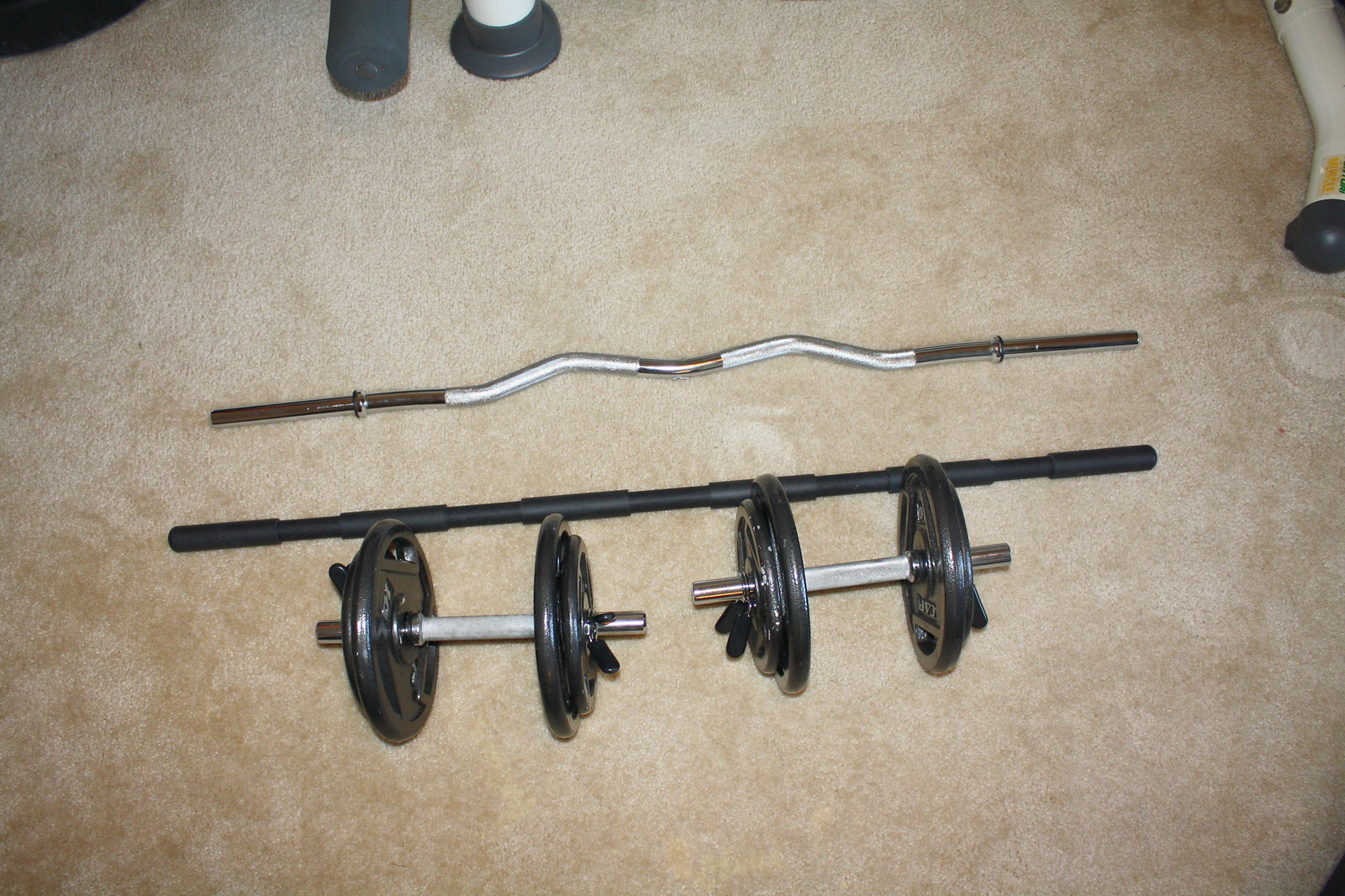This detailed color photograph shows various weightlifting equipment laid out on a textured beige carpet floor. At the top of the image, there's a long silver weight bar with a distinctive wavy middle section and straight, black ends that may have stoppers for securing weights. Below this bar, there is a second bar that is straight and black, with several notches or handle grips along its length. In the foreground, two sets of dumbbells are positioned next to each other. Each dumbbell features a glossy silver rod in the center and two black weights on each end, with one weight slightly larger than the other. Towards the top edges of the image, parts of other gym equipment are visible, including what appear to be metallic legs with grey, white, and black elements, and possibly a yellow sticker on one of them. The photograph captures a bird's eye view of the room, focusing on the contrast between the weightlifting equipment and the light beige carpet.